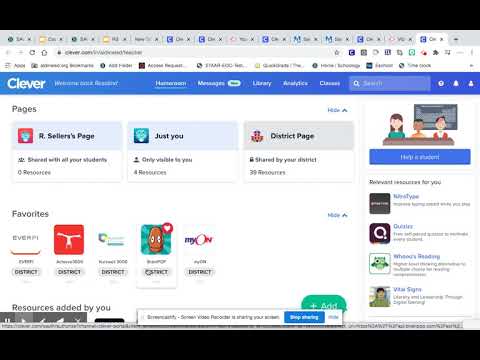This image appears to be a screenshot of a web browser, though the quality is quite low, making the text difficult to read due to its small size. The browser has multiple tabs open, with the current active tab being on the Clever platform. Within this tab, various clickable pages are visible, labeled as "R," "Serena's page," "Just You," and "District page." Additionally, there is a section titled "Favorites" displaying different icons.

At the top of the Clever interface, next to the company's logo, are several tabs labeled "Messages," "Library," "Analytics," and "Classes," accompanied by a search bar. Adjacent to the search bar are various icons, including a profile icon, a question mark icon, and additional indistinguishable icons. Near the bottom of the screen, partially cut off, a line of text reads "Resources added by you." The combination of these elements suggests a personalized educational dashboard or resource management tool.